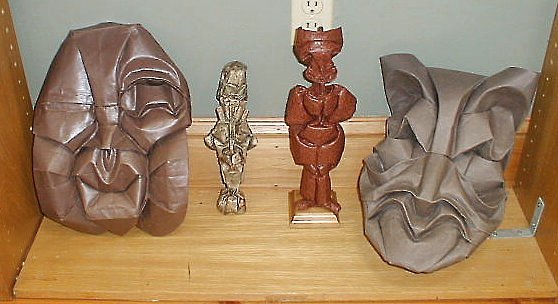The image showcases a lower wooden bookshelf against a light blue wall, with a power outlet visible in the background. Four distinct figurines are displayed on the shelf. On the far left, there's a copper-brown mask with a single eye opening, featuring a rounded, blob-like shape. Beside it, slightly to the right, is a gold-toned, nondescript statuette that is difficult to identify in detail. Further right is a reddish-brown figurine standing on a gold stand, facing the camera. Finally, on the far right, there is another mask, possibly made of metal or thick leather, with distinct facial features including ears, a nose, a mouth, and a chin. The arrangement and diverse materials of the figurines create a striking focal point against the blue wall backdrop.